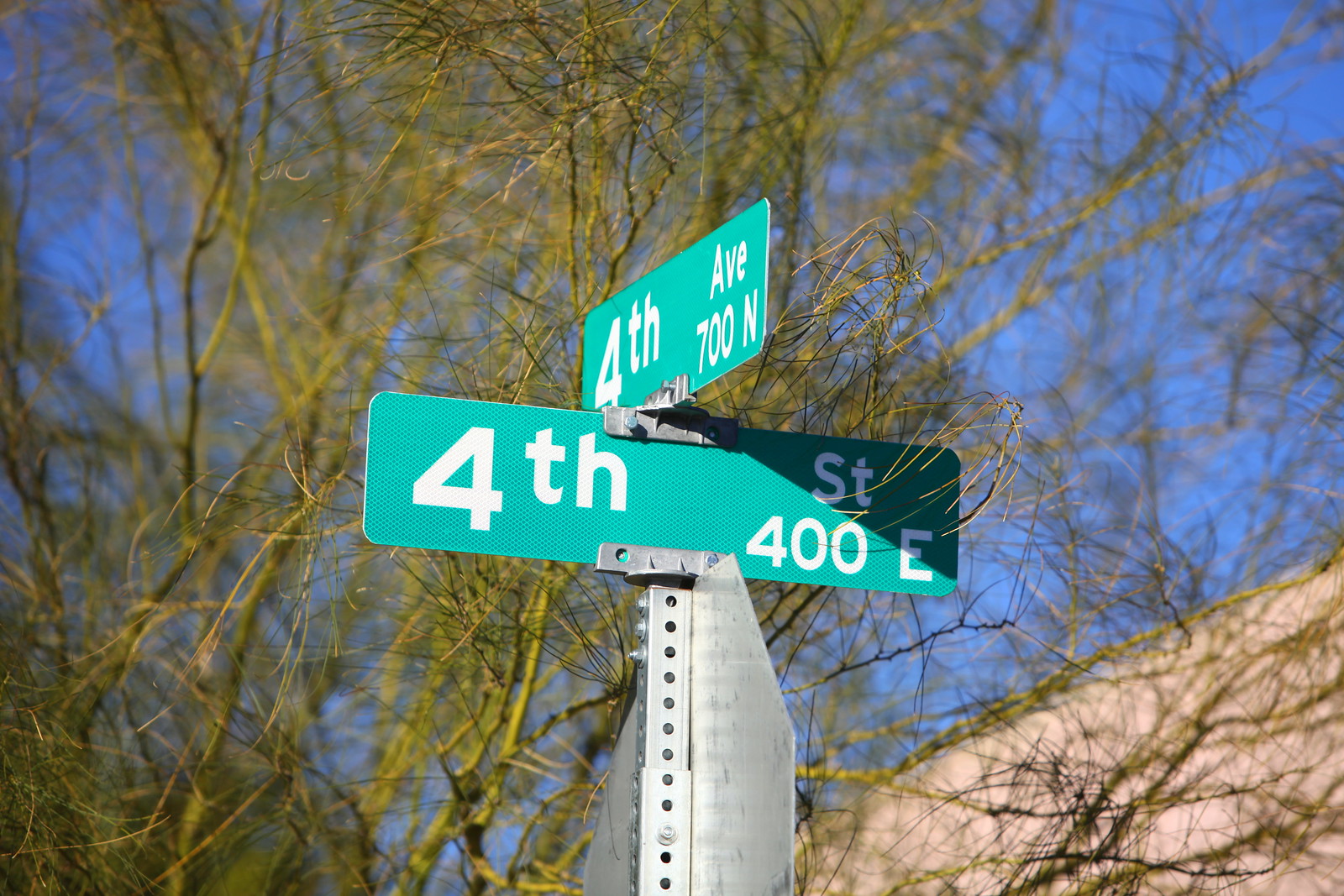The image frame is horizontally rectangular and captures an outdoor scene, focusing on the upper part of a street sign from a slightly upward angle. Dominating the composition is the back, silver-colored side of a stop sign, affixed to a steel post. Above the stop sign, two thin, rectangular street signs are mounted perpendicularly to each other. The lower sign, with a green background and white text, reads "4th Street, 400E." Directly above it, another green sign displays "4th Avenue, 700N." The backdrop includes a delicate network of very thin, almost hair-like branches stretching across.